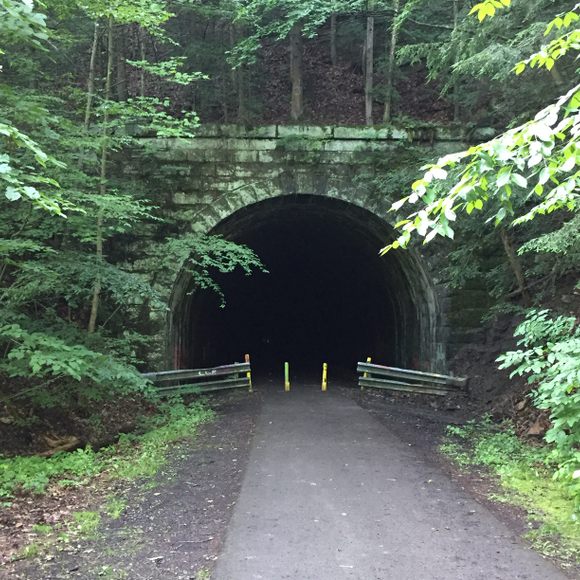The photograph captures an abandoned tunnel enveloped by nature within a dense forest. The tunnel, made of stone or concrete, is part of a bridge-like structure covered in green moss, adding a touch of mystique. Trees surround the scene, their branches arching over the top and both sides of the bridge, casting intricate shadows on the overcast day. In the foreground, a concrete pathway, bordered with a bit of grass, leads directly into the tunnel, which is partially blocked by metal fencing and traffic cones. The leaves on the trees nearby are dimly lit, suggesting an overcast day, and the humid environment is evident from the damp ground and lush moss. The dark, impenetrable interior of the tunnel contrasts starkly against the somewhat gloomy, yet richly green, forest setting.